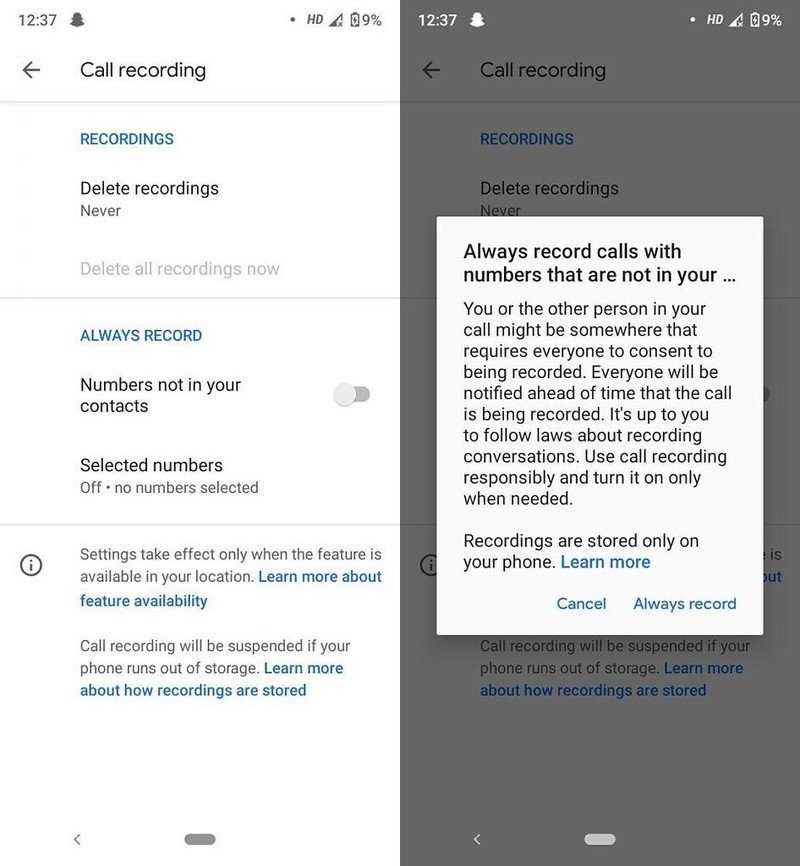The image consists of two side-by-side vertical mobile screenshots captured at 12:37 PM, each showing a battery level of 9%. The left screenshot features a predominantly white background, while the right one has a gray background with a white rectangle overlay.

### Left Screenshot:
At the top, the text "Call Recording" is displayed. Below that, the section title "Recordings" is highlighted in blue. The configuration settings include:
- "Delete Recordings: Never" 
- An option to "Delete all recordings now" is available.
- In blue, the option "Always record numbers that are not in your contacts" is present, with a slider pushed to the left, indicating that it is turned off. No numbers are selected.
At the bottom, there's a note stating, "Settings take effect only when the feature is available in your location." A blue hyperlink labeled "Learn more about feature availability" follows.
Further down, it is mentioned that "Call recording will be suspended if your phone runs out of storage," followed by another blue hyperlink, "Learn more about how recordings are stored."

### Right Screenshot:
The right screenshot includes an additional text box set against a gray background, titled "Always record calls with numbers that are not in your...". It provides detailed information:
- Notifies you that you or the other person on your call might be in a location requiring everyone's consent to be recorded.
- Everyone will be notified in advance that the call is being recorded.
- Emphasizes your responsibility to comply with applicable laws regarding recording conversations.
- Advises to use call recording responsibly and turn it on only when needed.
- Mentions that recordings are stored only on your phone.
A "Learn more" link is provided for additional information.

At the bottom of this text box, two clickable options are available:
- On the left: "Cancel"
- On the right: "Always record"

This comprehensive view highlights the settings and legal considerations of using the call recording feature on a mobile device.